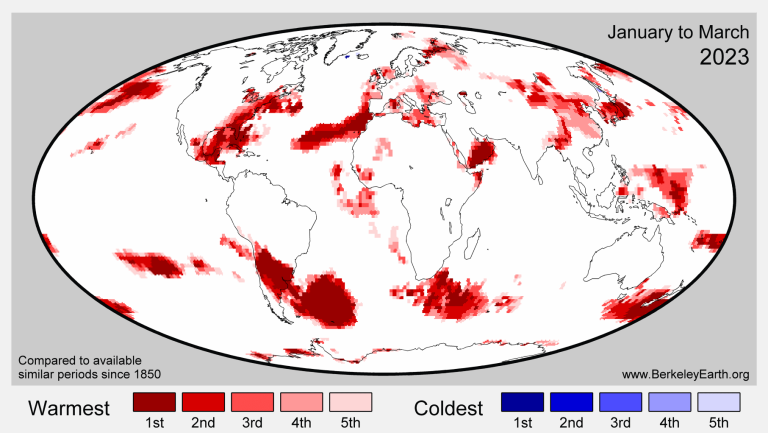This color image displays a world map in an oval projection, set against a grey rectangular background. Surrounding the map is a lighter grey rim on the top, left, right, and bottom edges. Below the map, black text labels "Warmest" and "Coldest" categories, each accompanied by five gradient rectangles ranging from dark red to pale pink (warmest) and dark blue to very light blue (coldest). Each rectangle is labeled first through fifth.

At the bottom left of the map, text reads "Compare to available similar periods since 1850," while the bottom right provides a URL: www.berkeleyearth.com. In the upper right corner, the date range "January to March 2023" is noted. A black oval line encircles the globe.

The map indicates the warmest areas primarily over the oceans near North Africa, Europe, the eastern coast of South America, the ocean southeast of Africa, the ocean just under and to the right of Australia, to the east of Russia, and between Russia and America. Notably, no blue areas (indicative of the coldest zones) are visible, suggesting a predominance of warmer temperatures during this period.